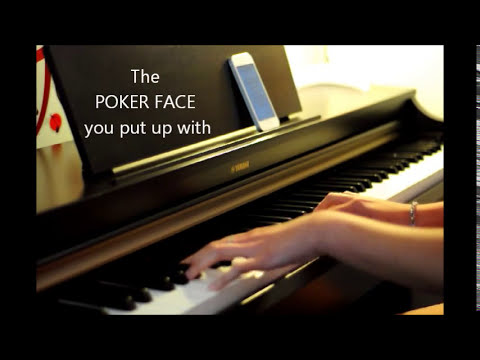The photograph shows a close-up of a person, likely a Caucasian woman, playing a Yamaha piano. Her hands, adorned with a bracelet on the right wrist, are positioned over the piano keys, actively engaging in playing a piece. The piano is black with white and black keys, and its name 'Yamaha' is clearly visible in gold lettering at the center above the keys. A white iPhone rests on the music stand, which has a black background featuring the words "the poker face you put up with" in white letters in the upper left corner. A small red musical note is noticeable against a white background near this text. The piano is partially open, and behind it, a white tablecloth with a red design is visible. The entire image is set within a dark, black and white frame, with a line of light reflecting on the right edge of the frame.